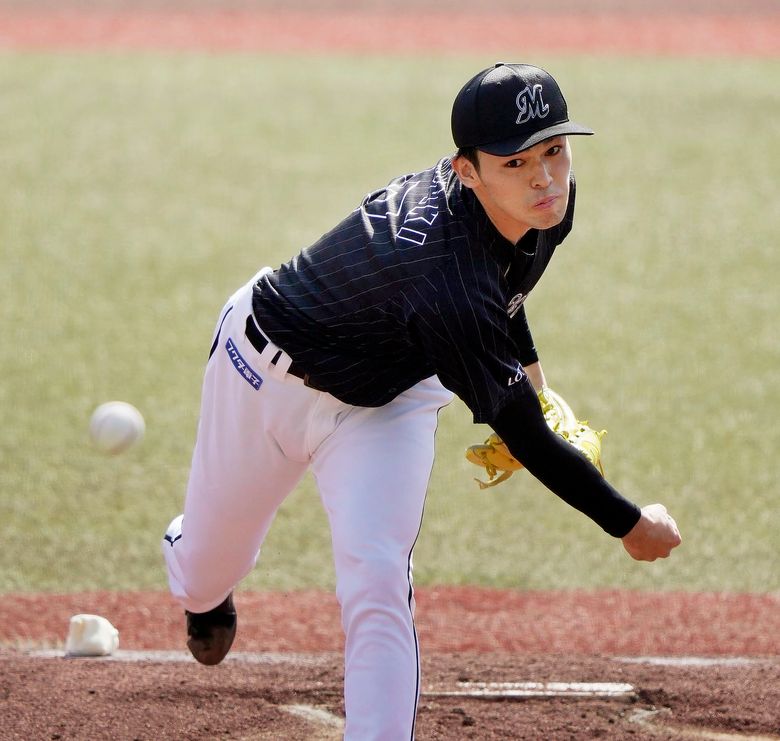In this detailed image, an Asian-looking young man, likely a teenager or young adult, is captured in the midst of pitching on a baseball field. The pitcher has black hair and brown eyes, and he is wearing a black baseball cap with a prominent "M" logo outlined in white. His black jersey features subtle white vertical stripes and white lettering on the back, covering his arms in full-length black spandex down to his wrists. His dynamic pose shows him leaning forward to the right after throwing the ball, which can be seen as a fuzzy blur to the left, continuing its trajectory towards the batter.

He wears white pants with a black belt, and a distinctive blue patch on the left side of his hip displays the numbers "7797" along with potential Japanese or Chinese characters. His shoes appear to be black. The pitcher's elevated mound is a dirt surface, with a small white base visible just below his shoe on the bottom left of the image. The background is mostly out of focus, featuring a light green field that subtly frames the action.